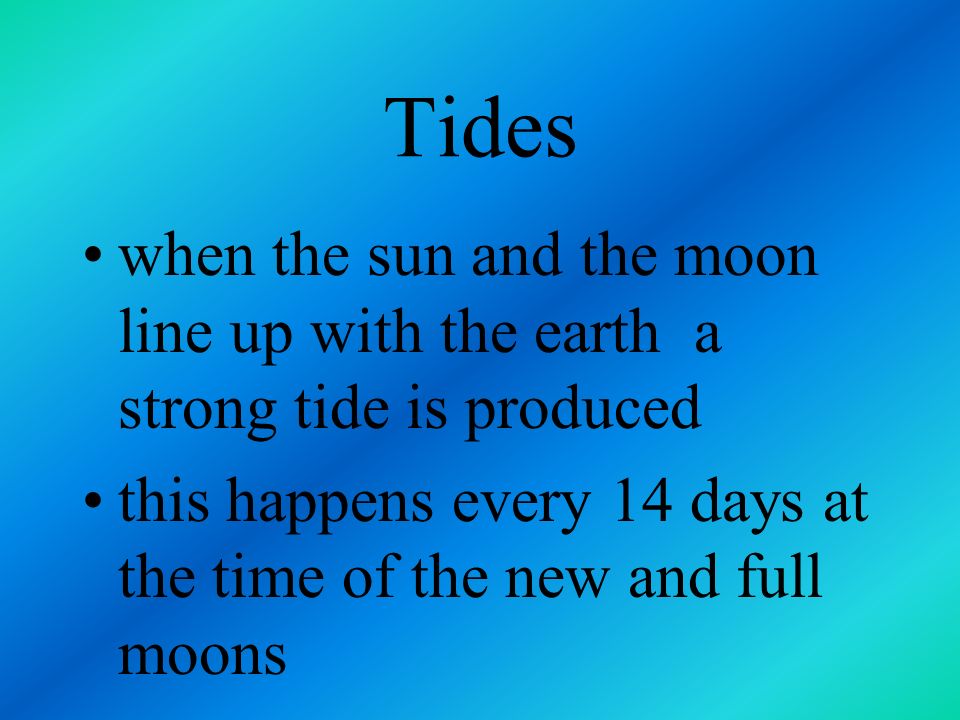The image is a PowerPoint slide with a gradient background that transitions from green in the top left and bottom right corners to a darker blue in the center. The background also features a faint diagonal stripe of darker blue running from the lower left to the upper right. At the top of the slide, centered, is the title "tides" in a slightly larger, non-bold Times New Roman font with a capital "T." The rest of the content includes two bullet points, also in black Times New Roman font, and all lowercase. The first bullet point states, "when the sun and the moon line up with the earth, a strong tide is produced," and the second bullet point reads, "this happens every 14 days at the time of the new and full moons." Notably, there is an extra space between the words "earth" and "a" in the first bullet point. There are no images present on the slide.